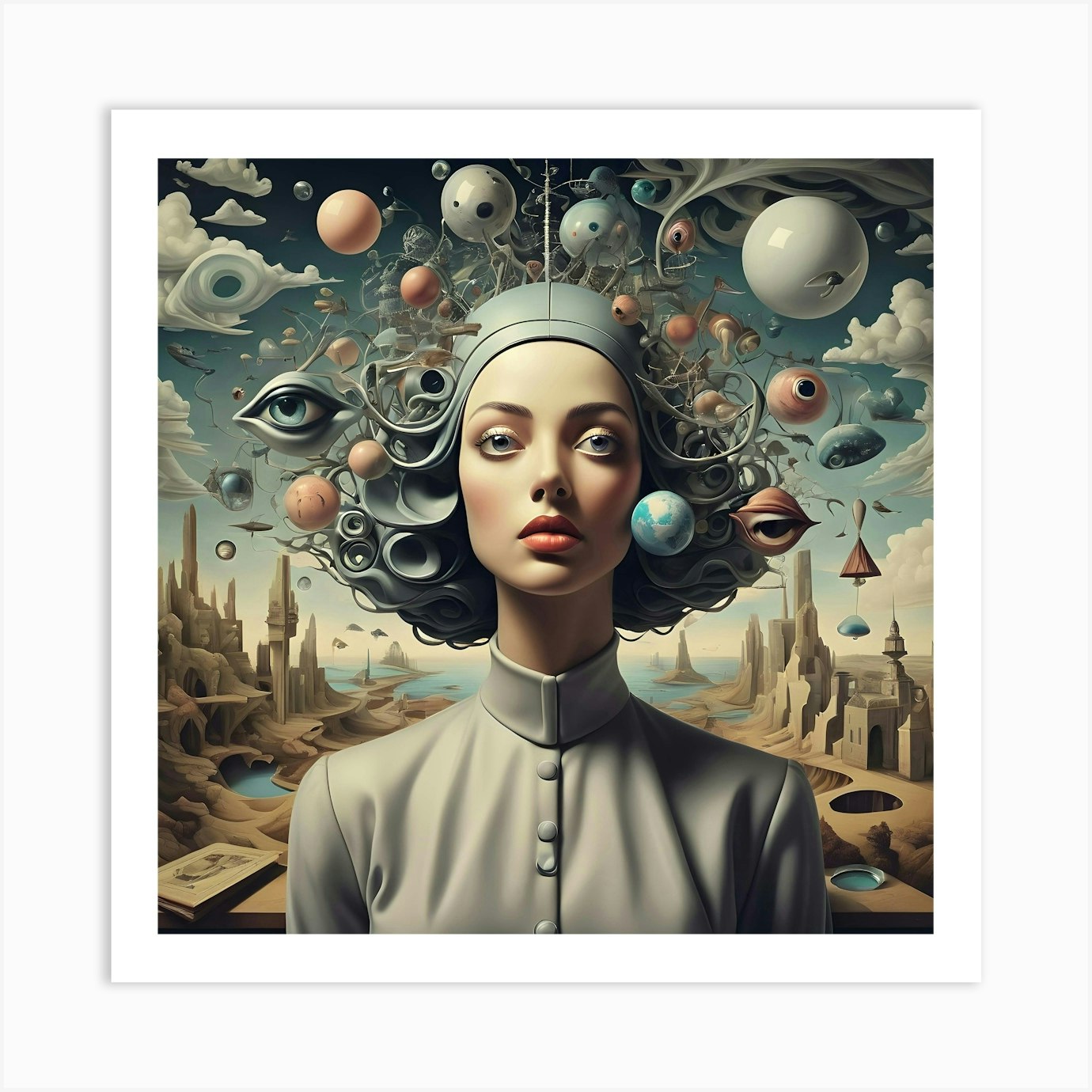The image is a stylized, futuristic painting of a woman staring straight at the viewer with a serene, composed expression. She wears a flowing blue hat with elaborate, curly, plastic-like extensions entwined with various floating spheres and eyeballs, some blue, some red, and some just black dots. The woman's long neck is encased in a high-collared, grayish-white top that features buttons down the front, conveying a modern, almost mystical aesthetic. Surrounding the hat are white fluffy clouds and additional spherical shapes that resemble planets or celestial bodies. 

The background combines an intriguing mix of natural and urban elements: a desert-like cityscape with earthy, sand-colored structures of varying heights dominates the left and right edges of the scene. On the left side, a small pond sits in front of the buildings, while on the right, there is an empty pond, adding to the surreal atmosphere. Directly behind the woman, a vast sea stretches out to meet the skyline, highlighting the vastness and the seamless blend between the earthly and the otherworldly. Additionally, to her left, there's a table with a book, further enriching the narrative complexity of the artwork.